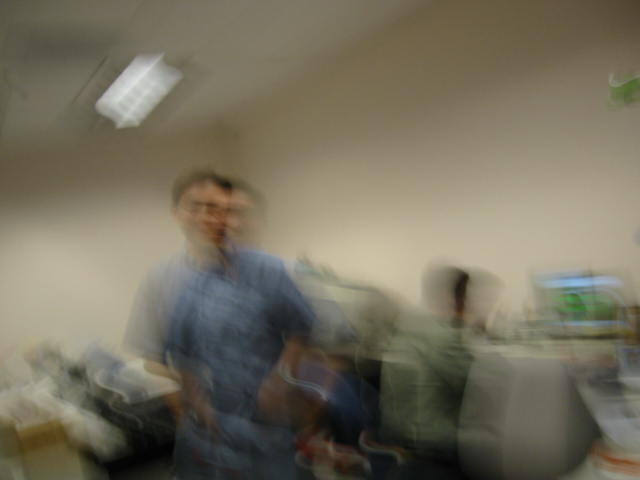A very blurry photograph captures a young man standing in what appears to be an office space with white walls. The room features a white-tiled ceiling illuminated by a fluorescent office light. The man, who has white skin and dark brown hair, is dressed in a slate blue short-sleeve t-shirt and glasses. He is looking at the camera, smiling, with both arms bent at the elbows and his hands raised slightly in front of him. In the background, an office chair with a blue seat and silver frame is visible. Other objects are aligned along the wall and on a table behind him, though they are too blurry to distinguish.